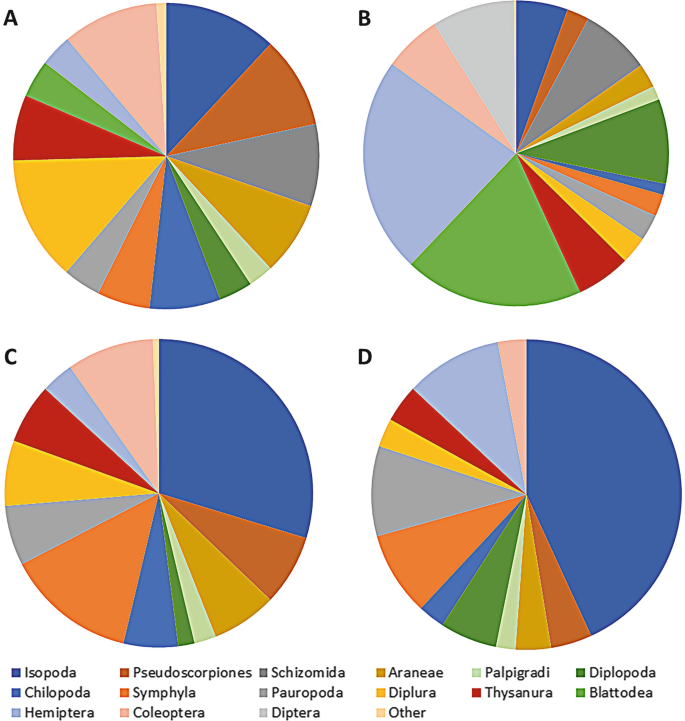The image features four distinct pie charts labeled A, B, C, and D, arranged in a grid with A at the top left, B at the top right, C at the bottom left, and D at the bottom right. Each pie chart is vibrant and colorful, featuring segments in various shades including blue, light blue, very light blue, orange, yellow, green, light green, gray, brown, pink, and red. These colors represent different categories, as indicated by a legend located below the charts. For instance, dark blue represents Isopoda, lighter blue denotes Chelopoda, and very light blue signifies Hemiptera. Other colors such as brown, orange, and pink correspond to categories like Pseudoscorpions, Symphyla, and Coleoptera, respectively. The image has a white background and the text is written in black, ensuring clear readability under natural lighting conditions.